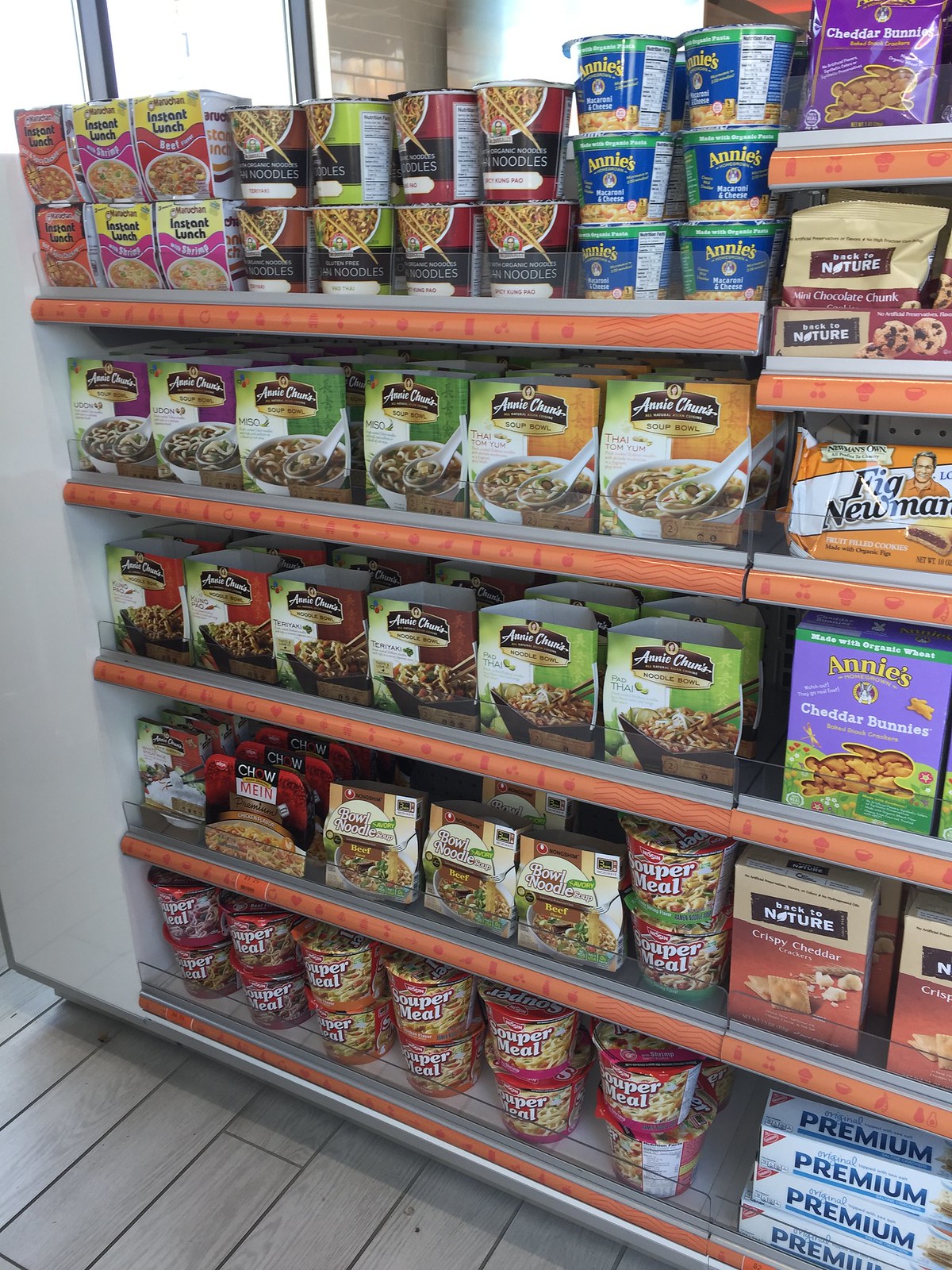The image depicts a brightly lit section of a small grocery store, focused on an aisle brimming with various food products. The shelving, which features a distinctive orange or red plastic edging, is impeccably organized with no gaps where products have been removed. Each shelf, five in total, is filled with different items, predominantly showcasing instant soups and crackers.

On the top shelf, there are numerous packages of instant noodles, including recognizable brands like "Instant Lunch" and "Bowl Noodle," showing images of white bowls with forks twirling up noodles. Below this, particularly on the second shelf, there's a box labeled "Back to Nature" with crispy cheddar crackers, and more containers of a product labeled "Super Meal," clearly spelled as s-o-u-p-e-r.

The bottom shelf features a white box with blue lettering that says "Premium" prominently on the side. Next to it, there's another set of containers for "Super Meal" that look like plastic bowls. To the left end of the shelves, an end cap is visible, standing out with its white color, and the floor below is made of light gray artificial wood planks. Both the edges of the shelves and the walls at the end of the aisle are white, contrasting the vibrant packaging colors.

Numerous brands repeat throughout the shelves in different sections, suggesting a healthy variety such as "Cheddar Bunnies" and cereals, possibly including muesli. Overall, this meticulously arranged section gives a clear and detailed view of the organized and diverse range of snack foods and instant meals available in this small supermarket.